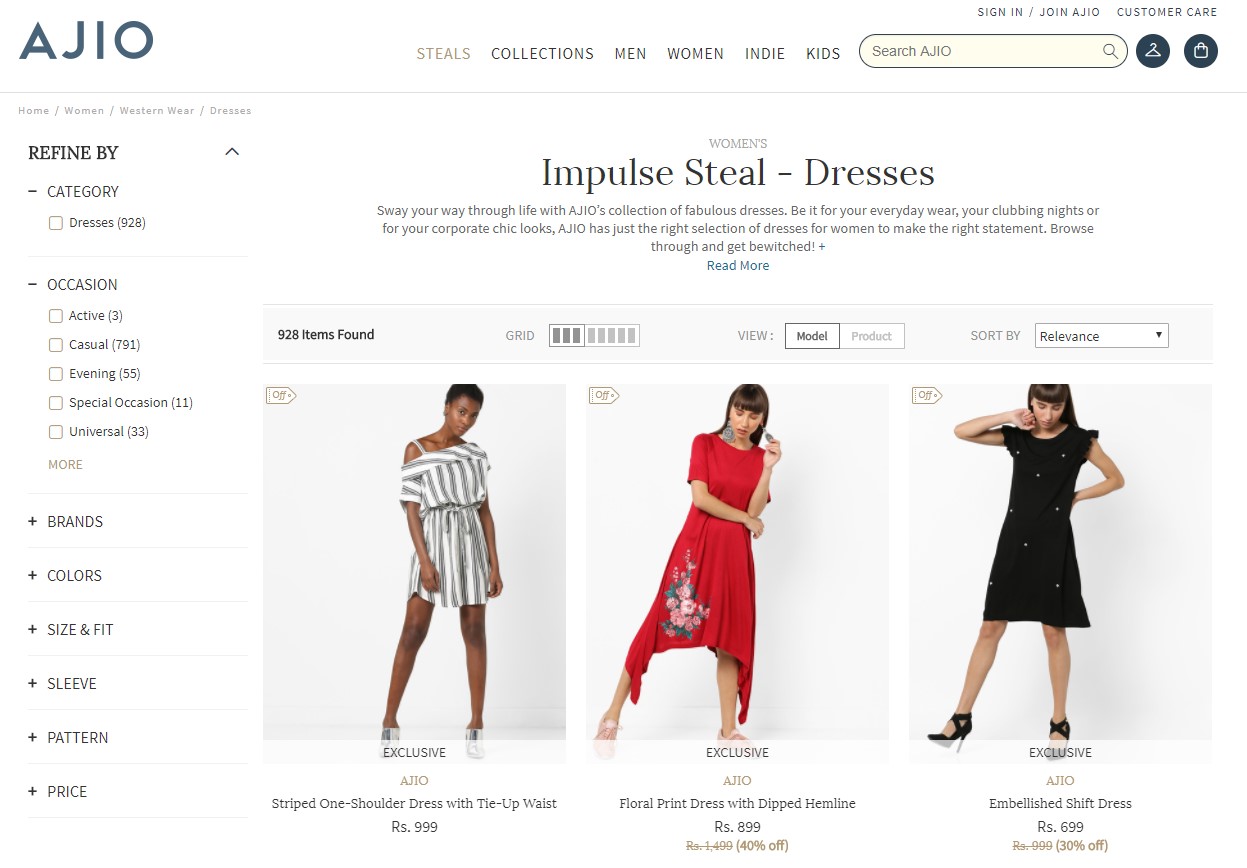This is a detailed photograph of the Ajio website, prominently displaying its women's clothing section. Ajio, spelled A-J-I-O, offers a variety of categories listed at the top of the page: Steals, Collections, Men, Women, Indie, and Kids. The navigation bar also includes a search function, options to sign in or join Ajio, customer care access, and a shopping bag icon accompanied by a hanger emoji, whose exact purpose is unclear but may imply a try-on feature.

In this image, under the 'Women's' category, the focus is on 'Impulse Steal' dresses, with three distinct dresses featured:
1. A gray and white striped one-shoulder dress with a tie-up waist, which has a romper-like appearance.
2. A red dress with short sleeves, adorned with floral detail. This dress features a high-low hem with the sides being longer than the front and back.
3. A black dress with frilly short sleeves and white polka dots, paired with black shoes.

The website offers extensive filtering options for refining dress searches by occasion (active, casual, evening, special occasion, and universal), as well as by brand, color, size and fit, sleeve type, pattern, and price range.